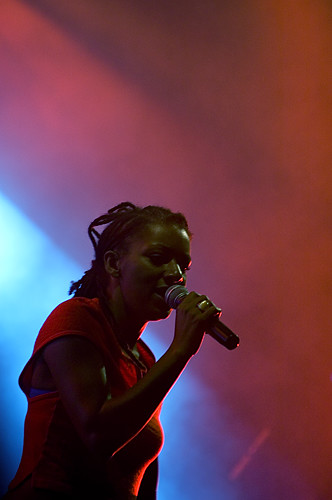The image captures a close-up of a young black woman with braided hair, appearing to perform on a stage. She holds a handheld microphone to her lips, wearing a deep orange or red form-fitting top, with a large ring on the fourth finger of her right hand. The image is taken from the waist up and framed vertically. She emerges from the lower left corner, occupying the central portion of the photograph. The background presents a dark setting, possibly a nightclub or bar, with shafts of stage lighting and an out-of-focus tarp or tent roof above her. Blue and green lights emanate from behind, mingling with orange hues from above, creating a vibrant, atmospheric scene filled with smoke that scatters the light. The composition of lighting and smoke adds depth and mood to the performance moment captured.